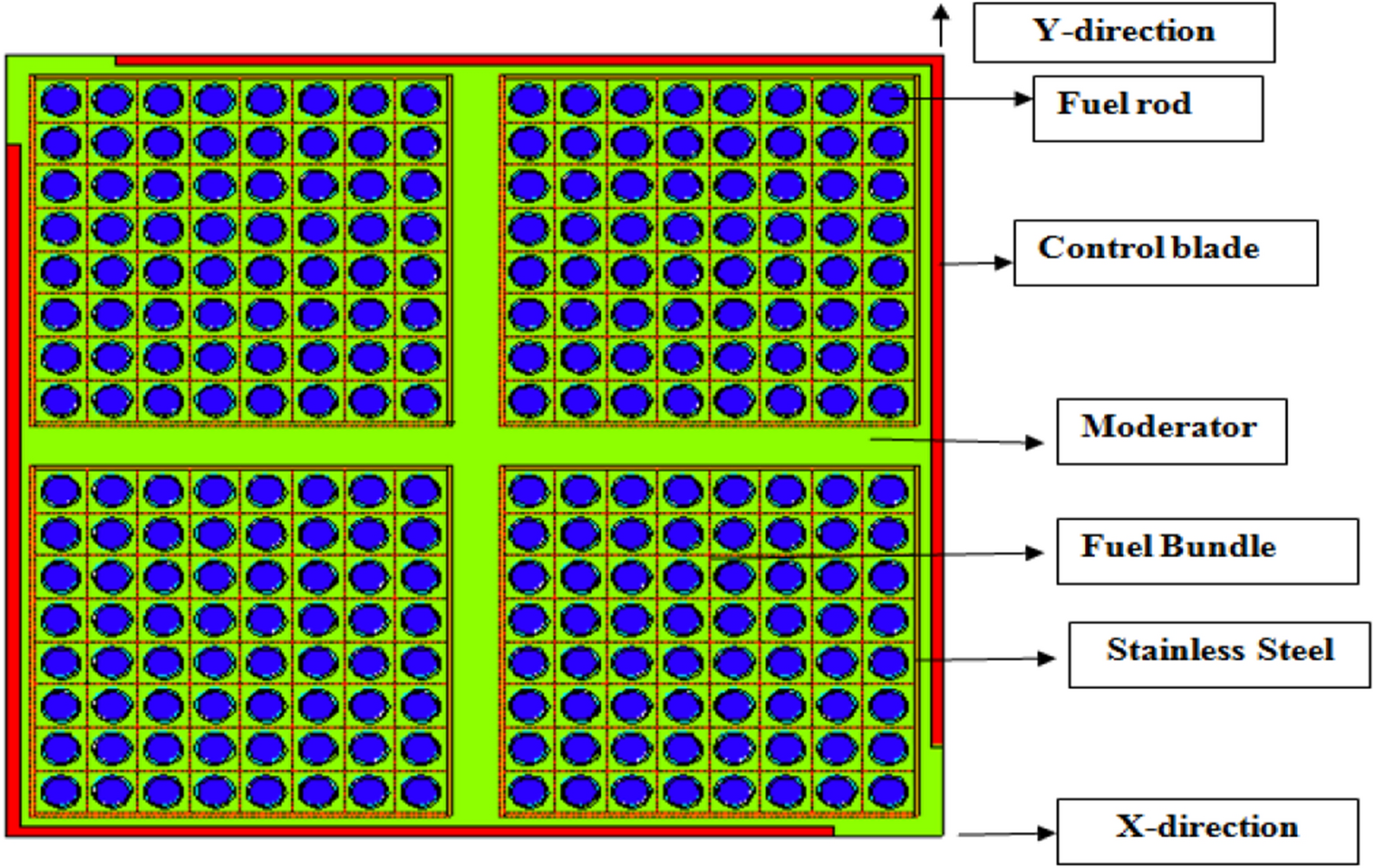This image features a large square on a solid white background, prominently bordered in red except for the upper left and lower right corners where the border is green. Within the large square, there are four smaller squares, each containing an 8 by 8 grid of blue circles, making 64 circles per square. These smaller squares are separated by a thick, neon green cross shape, creating four distinct quadrants. Black arrows point rightward from the squares leading to text boxes, which read, from top to bottom: "Y direction" (with an up arrow), "Fuel rod," "Control blade," "Moderator," "Fuel bundle," "Stainless steel," and "X direction" (with a right arrow).